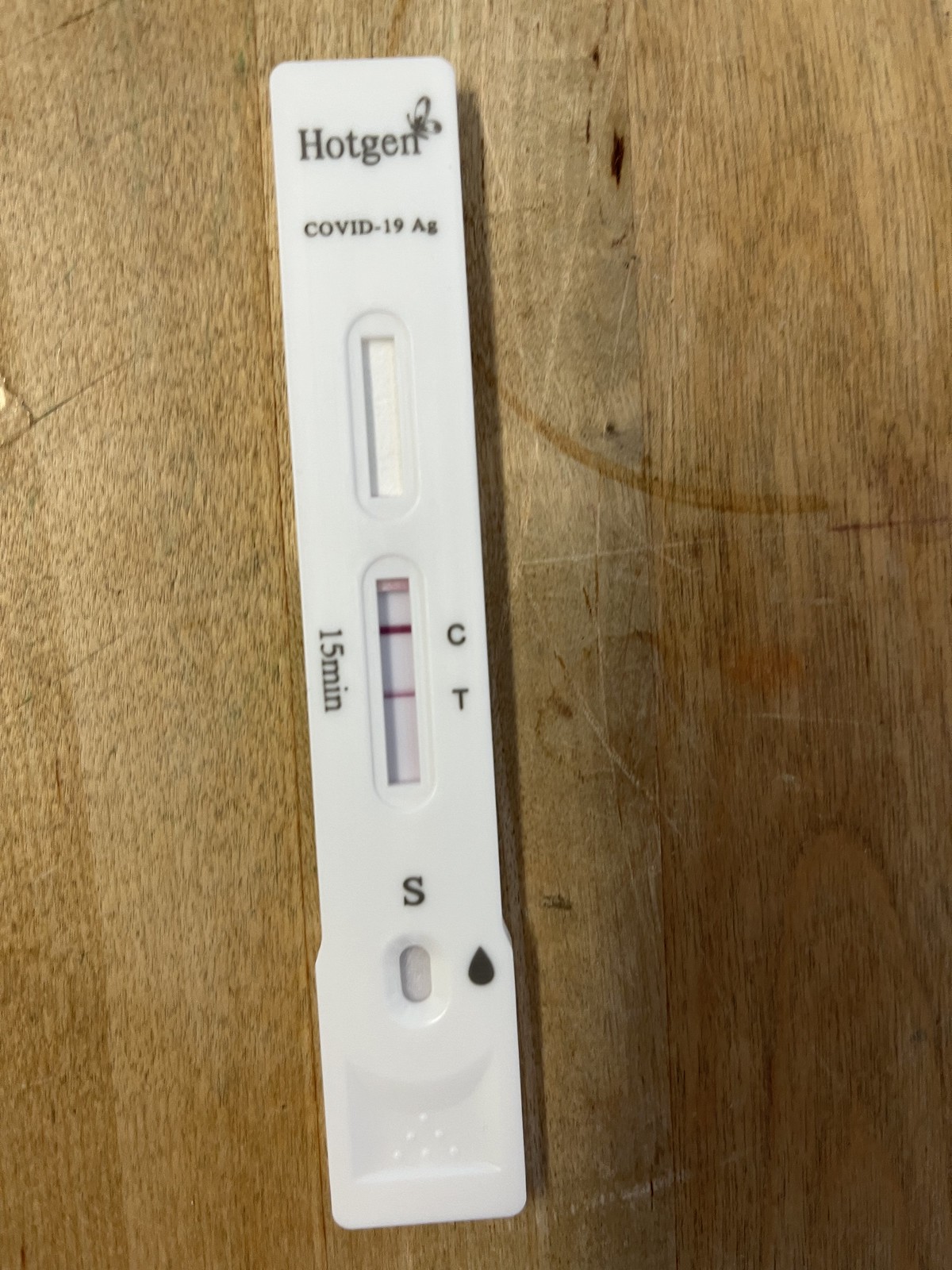This photograph captures a completed COVID-19 rapid test kit, prominently displaying a positive result on a scarred wooden table. The test device, made of white plastic, bears the brand name "Hotgen" and features two lines labeled "C" and "T," both of which are filled in, indicating a positive diagnosis for COVID-19. The 15-minute test appears to have been carefully timed, and the photo seems to have been taken after the result was confirmed, possibly to share the outcome on social media. The test kit shows the designated spot for depositing the test liquid, prepared after swabbing, illustrating that all necessary steps to conduct the test were meticulously followed.